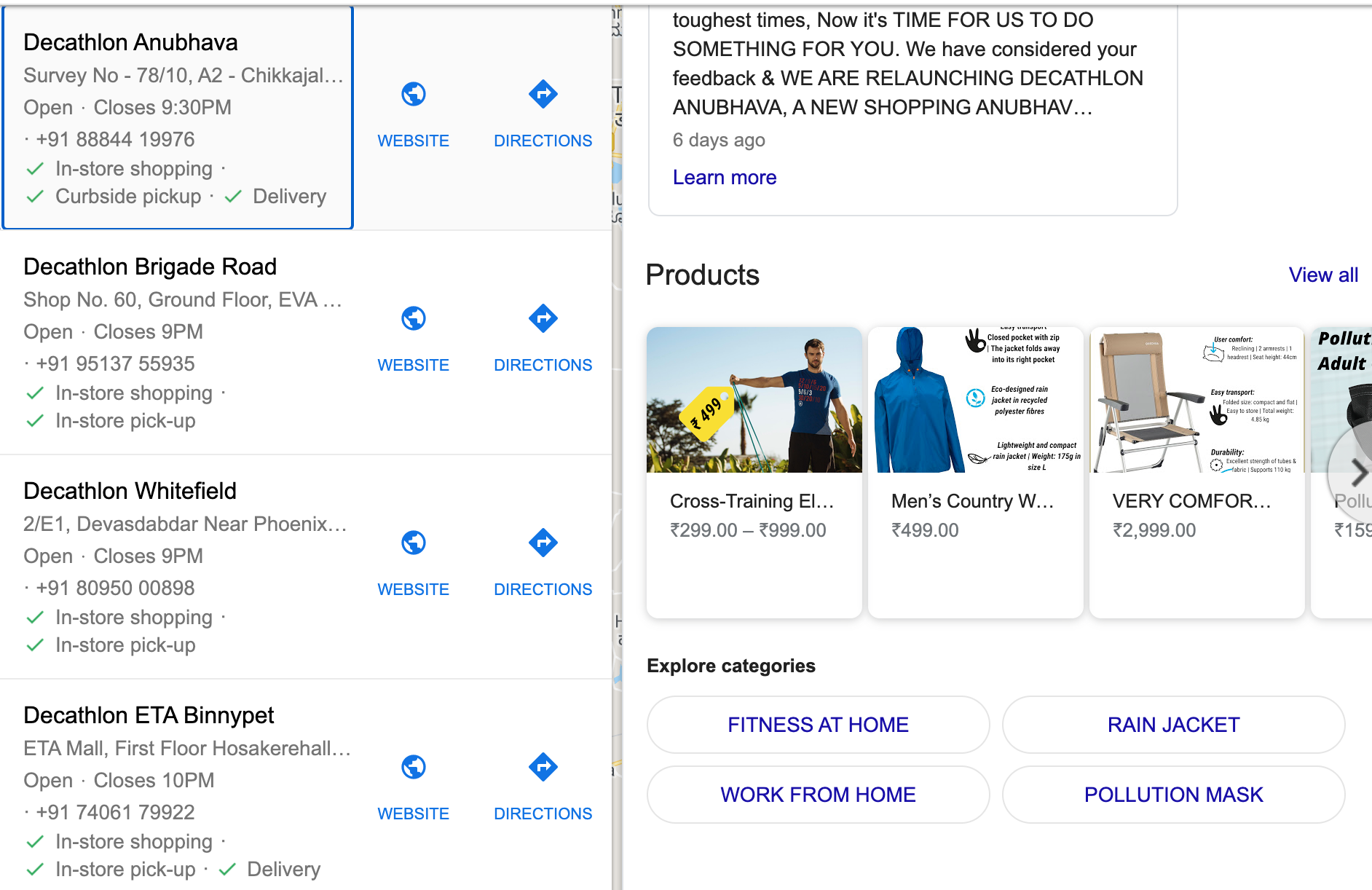The image depicts a detailed advertisement for a Decathlon store in India, possibly the Whitefield branch. The top left corner prominently features the Decathlon logo alongside another logo resembling that of Barack Obama. Below these logos, there's an array of store-specific information, including operational hours—indicating the store closes at 9:30 PM—and service options like in-store shopping, curbside pickup, and delivery.

A segment of the text specifies the store's exact location on Bridget Road, highlighting both onsite and delivery services. The bottom part of the image provides web links and directions for added convenience. On the upper right section of the image, there is skewed text outlining a recent relaunch of Decathlon's new shopping experience, accompanied by a product promotion for men's country gear priced at 2,999 INR.

The image also encourages exploring various categories such as fitness equipment for home use, rain jackets, work-from-home essentials, and pollution masks, ensuring a comprehensive shopping experience for diverse customer needs.